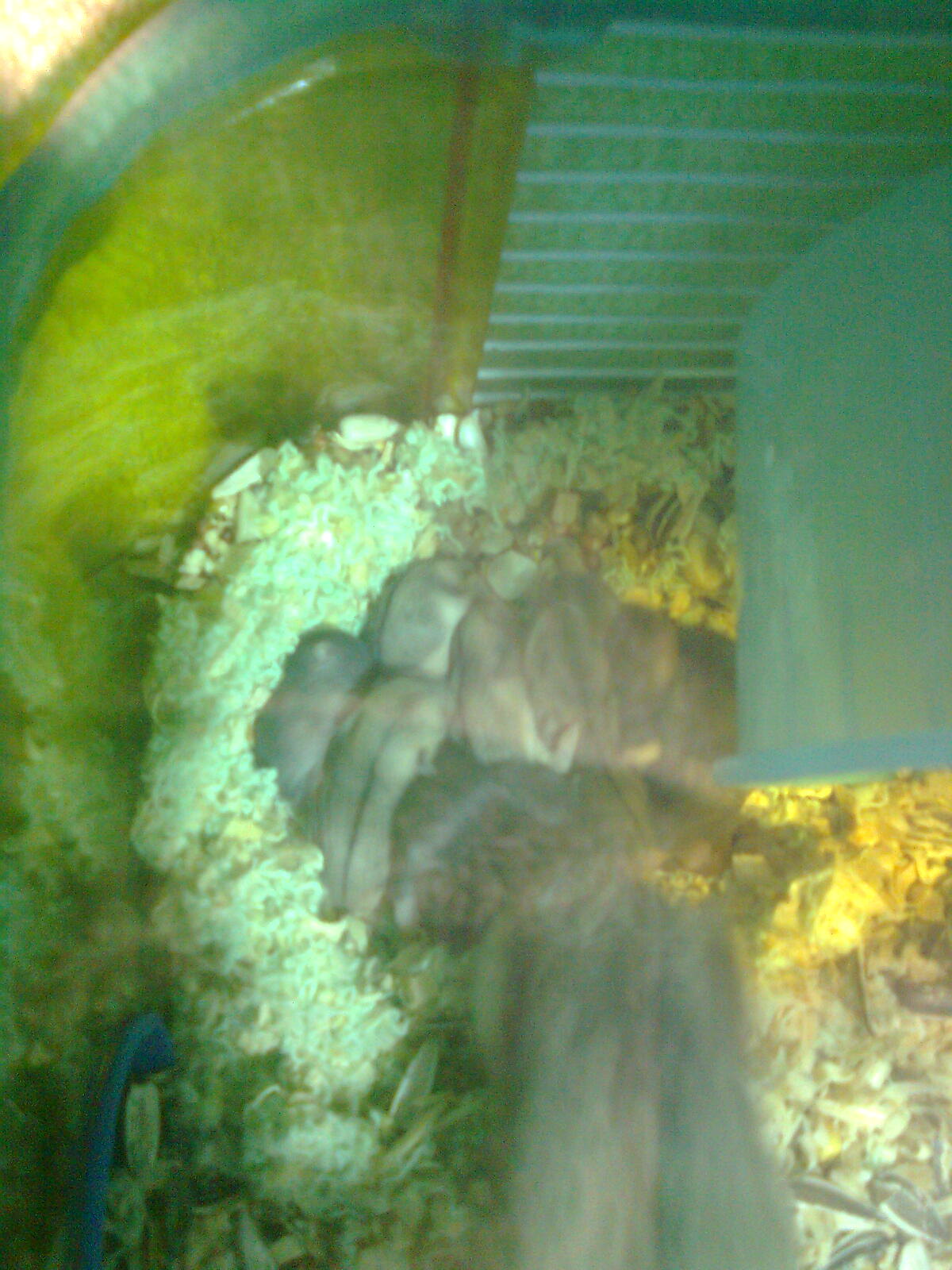The somewhat blurry color photo shows a group of tiny, newborn hamsters nestled together in the center of a hamster cage. The delicate pile of brown, furry baby hamsters appears to be sleeping on a bed of shredded straw or hay-like bedding, with bits of sunflower seeds and hamster food scattered around them. Positioned in the bottom center is the larger figure of the mother hamster, partially visible but tending to her litter. To the right, a blue plastic hamster wheel and a blue heat lamp emitting a yellow light can be seen, casting a reflective glow across the cage's rounded, see-through walls.